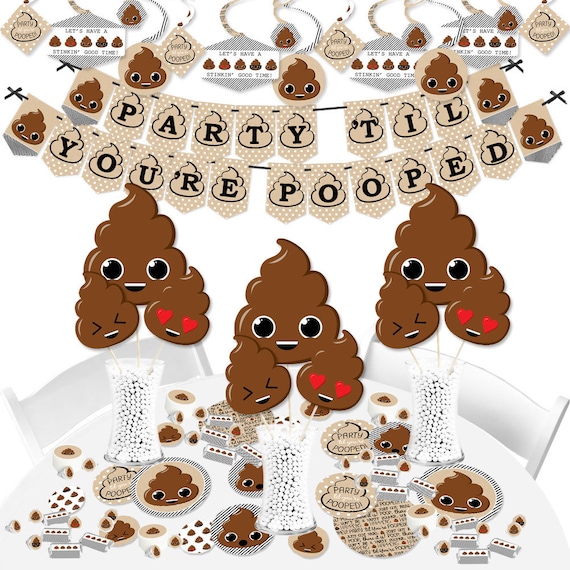The digitally created image displays a vibrant, poop emoji-themed party setup. Central to the composition is a white table adorned with various poop emoji decorations, including large poop figures. These emojis display different expressions, such as heart-shaped eyes, grins, and closed eyes, and are arranged in flower holders filled with white beads. Positioned on the white table, these decorations are improbably flat against an angled surface, suggesting a photoshopped composition. The backdrop is a clean, white setting featuring white chairs.

Above the table is a prominent banner with the phrase "Party till you're pooped," flanked by more poop emojis and smaller banners echoing the same text alongside "Let's have a stinking good time." The emojis are primarily brown, with accents of black and red for eyes, set against white and gray tones in the backdrop.

The overall style is that of a promotional display image, possibly an advertisement for party decorations or favors, emphasizing a playful and quirky theme. The setup includes a mixture of text and imagery, creating an inviting, albeit surreal, party atmosphere.